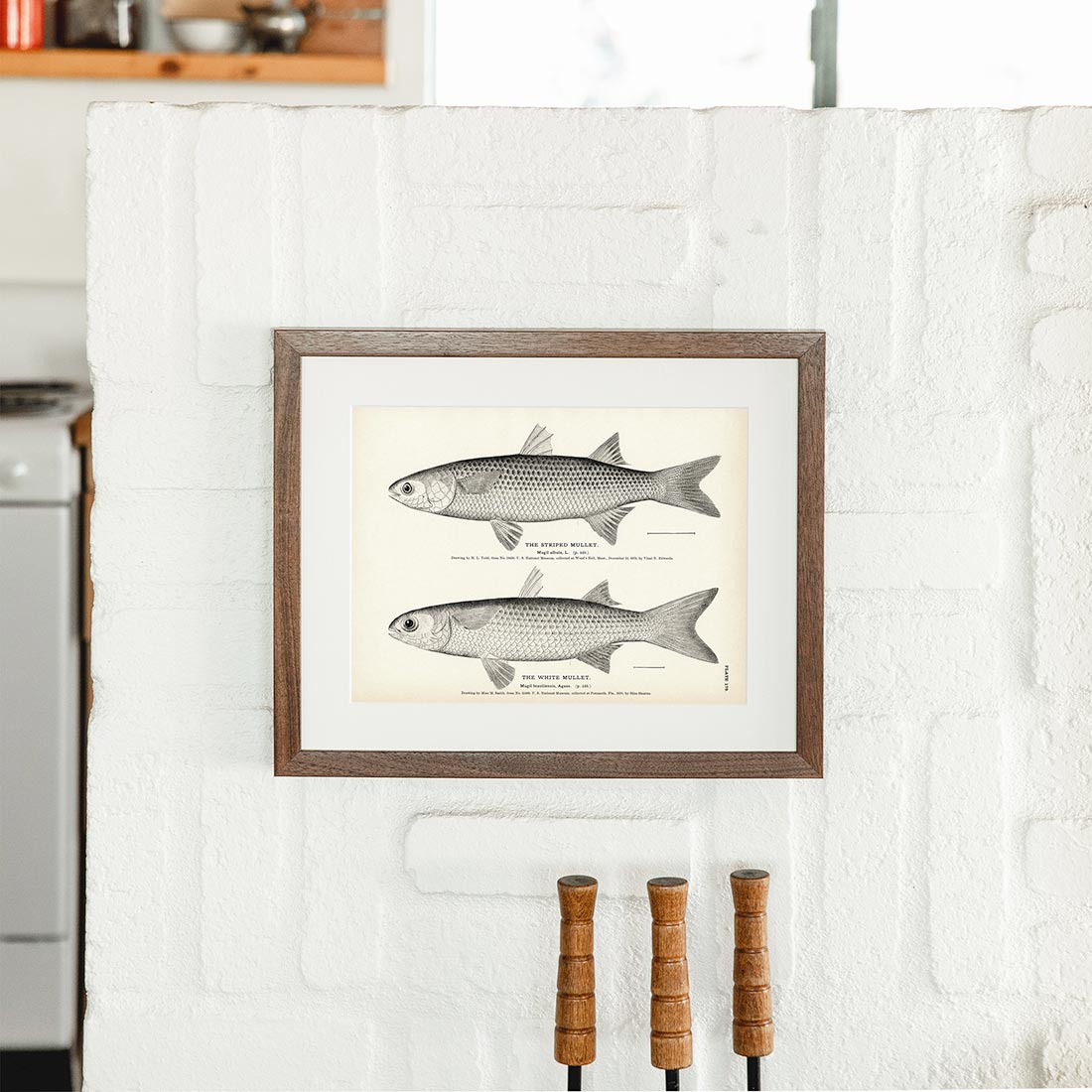In the photograph, there is a well-framed wood picture mounted on a distinctive wall, which appears to be composed of uniquely arranged bricks, alternating between three upright and three horizontal. The framed picture features detailed black-and-white drawings of two fish, one positioned above the other, and is labeled with their types. The image is situated in a kitchen, evidenced by the visible stove and shelving with pots above it. Below the fish drawing, there are three handles, likely for kitchen or fireplace tools. The overall setting suggests a rustic kitchen ambiance with a close-up view of part of the kitchen space, highlighting the eclectic and functional decor.